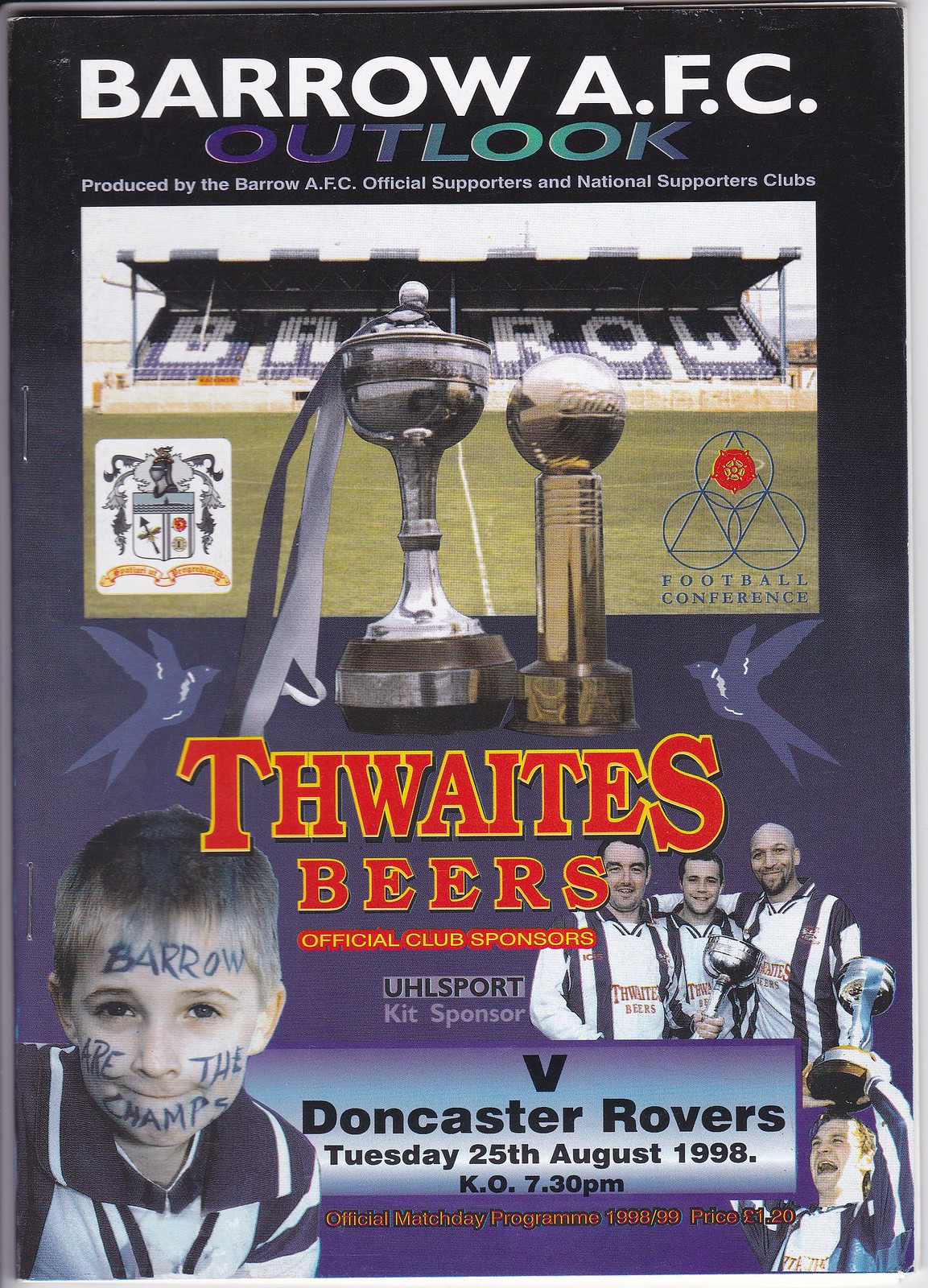The flyer for Barrow AFC Outlook, presented on a page with the dimensions akin to a magazine, features a striking purple background with "Barrow AFC" in white text at the top, transitioning to "Outlook" in purple-to-green gradient text. An image of Barrow's small stadium graces the cover, showcasing a row of covered bleachers with "Barrow" emblazoned on the seats and a clear view of the field.

Prominently displayed in the center are two trophies, with bold red and yellow-outlined text underneath proclaiming "Thwaites Beers, Official Club Sponsors." Also noted is the UHL Sport kid sponsor. On the lower left, a photograph captures a child with "Barrow, the champs" painted on his face. The lower right quadrant features celebratory scenes: a group of three men in football jerseys holding a trophy and a solitary man triumphantly lifting a trophy above his head.

Additionally, the flyer details an upcoming match: "Barrow AFC Outlook vs. Doncaster Rovers, Tuesday, 25th August 1998, KO 7:30 p.m., official matchday program 1998-99, price £1.20."